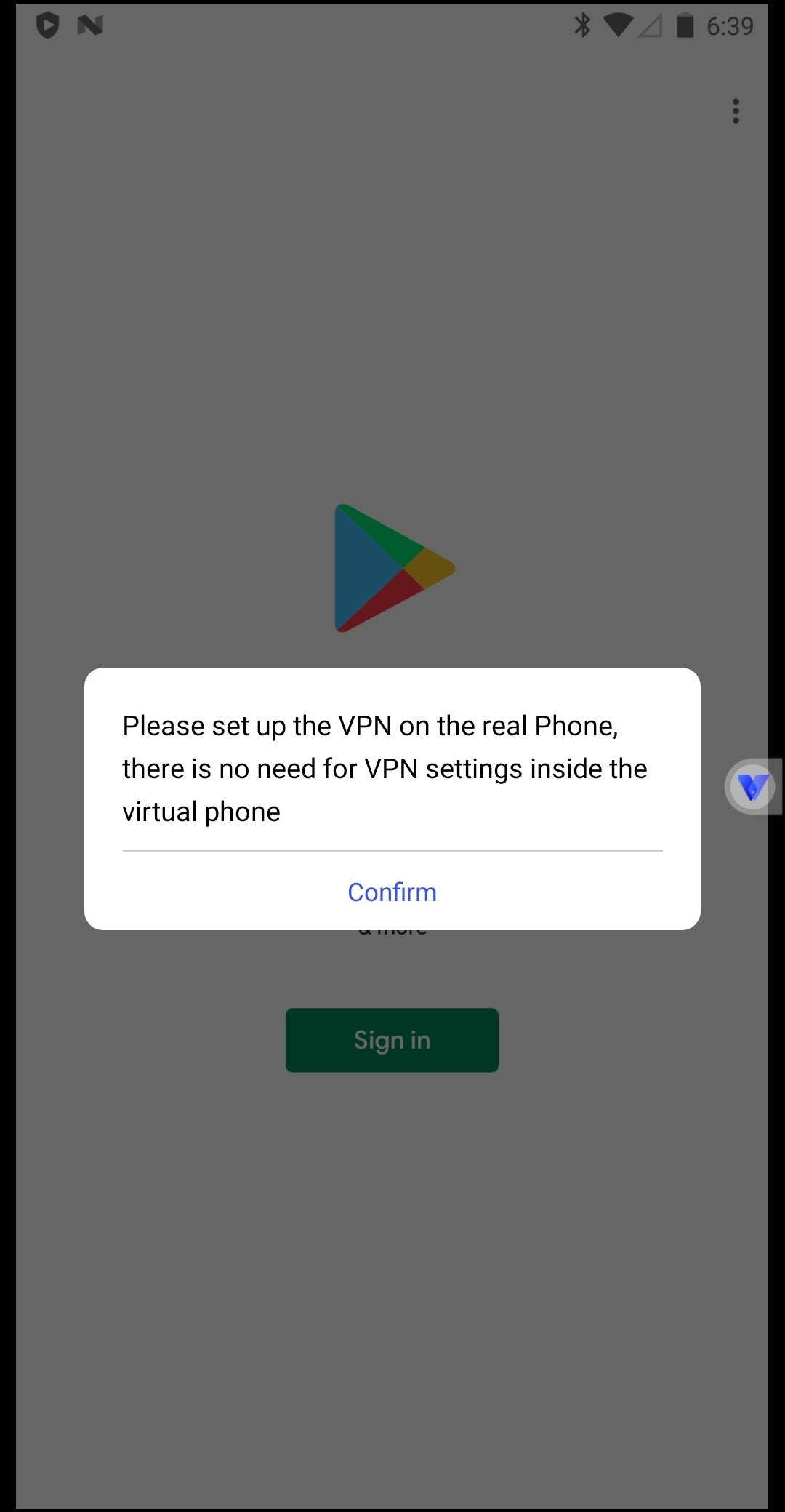An Android phone displays the Google Play Store in the background, featuring a prominent pop-up requesting user action. The pop-up, adorned with the Google Play Store logo, prompts the user to "Sign In" through a conspicuous green button. Below the button, an informational message reads: "Please set up the VPN on the real phone. There is no need for VPN settings inside the virtual phone," followed by a clickable "Confirm" option.

In the notification bar at the top of the screen, several icons are visible, giving additional context to the phone's status. On the left, a shield icon, likely representing a security app, is accompanied by what appears to be the NerdWallet logo. To the right, symbols for Bluetooth, Wi-Fi signal strength, mobile data signal strength, battery level, and the current time, 6:39, are displayed. This meticulously detailed screenshot captures the intricacies of an Android user's interface, highlighting the interplay between app functionalities and system notifications.